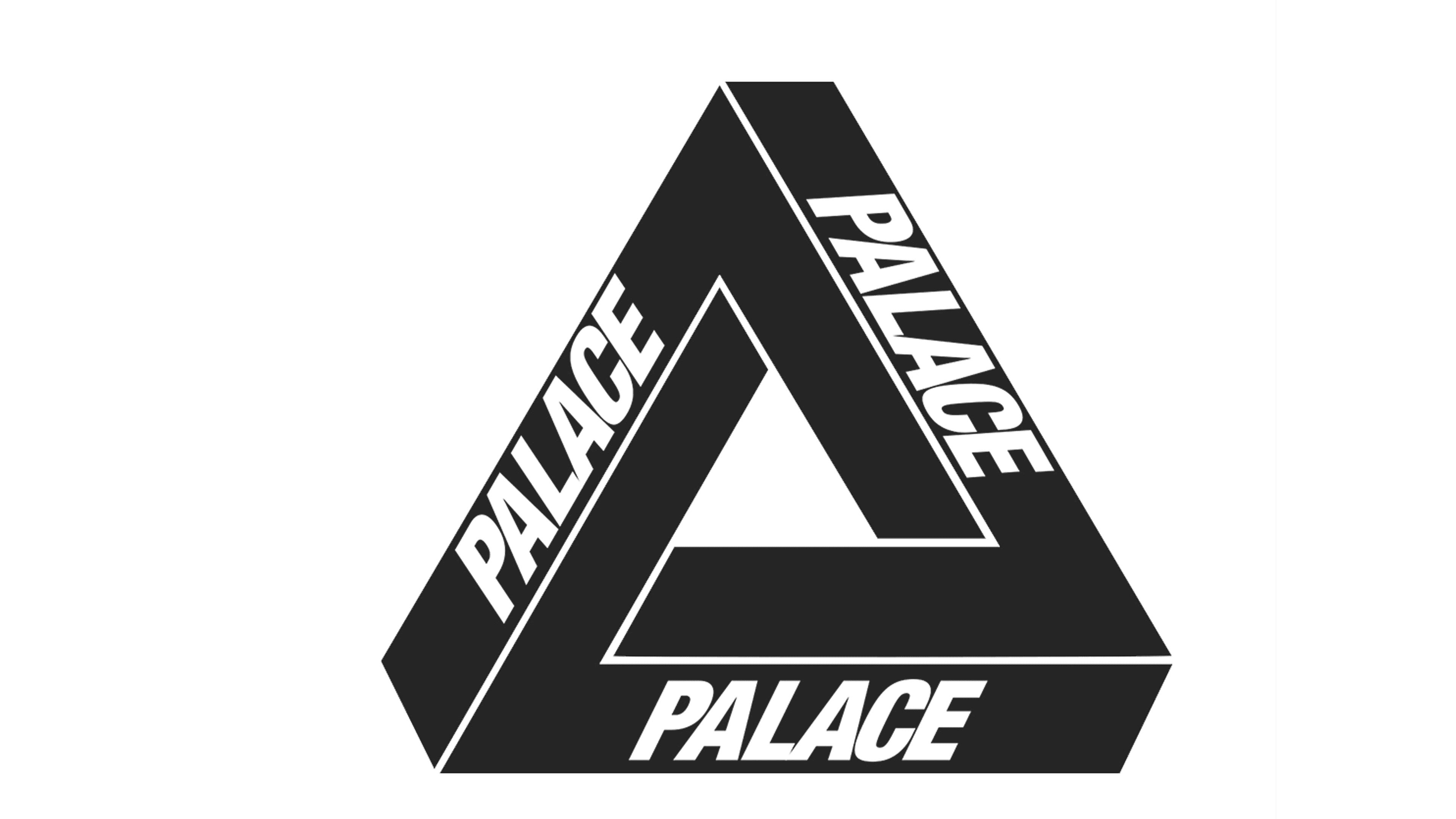This image features a black triangular logo for a company named Palace. The design is an optical illusion resembling a 3D Penrose triangle, which appears perfectly triangular from the front but reveals its impossibility if viewed from an angle. The triangle has square edges rather than pointed corners, creating a unique visual effect. Each side of the triangle prominently displays the word "Palace" in bold, white block letters: one side displaying it vertically, another horizontally, and the third diagonally. The interior of the triangle is left empty, further emphasizing the clever use of perspective to portray the logo as a cohesive, albeit impossible, shape.